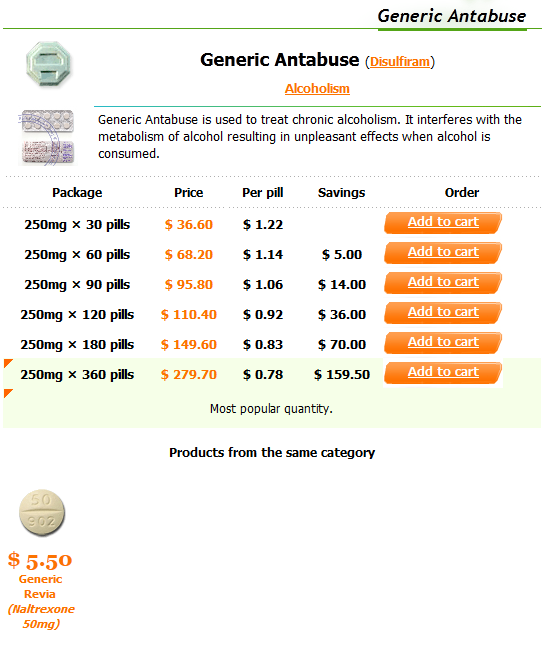The image features a detailed advertisement for Generic Antabuse, a medication used to treat chronic alcoholism. 

In the top right corner, the headline "Generic Antabuse" is prominently displayed in black with a green underline. Below it, the text repeats "Generic Antabuse," this time followed by "Disulfiram" in orange parentheses. The word "Alcoholism" appears in orange below this.

On the left side of the image, a green pill with a wide letter "A" symbol is shown. Underneath, a description explains that Generic Antabuse is used to treat chronic alcoholism by interfering with the metabolism of alcohol, resulting in unpleasant effects when alcohol is consumed. Several pills are also depicted, encased in silver blister packaging.

The lower section of the image presents a chart listing different package sizes, prices, and savings. For example, 30 pills of 250 milligrams each are priced at $36.60, with prices increasing as the quantity goes up, reaching $279.70 for the largest package. The per pill prices and savings are also displayed. An orange "Add to Cart" button invites users to place an order, and a "Most Popular Quantity" note enhances the call to action.

At the bottom, the section "Products from the Same Category" highlights another medication, showing a pill labeled "50" and "902" with the name "Generic Revia." This adds an additional option for consumers seeking alcoholism treatment.